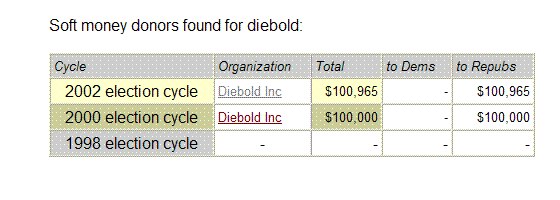The image contains a graph titled "Soft Money Donors Found for Diebold," detailing contributions made by Diebold Inc. across three election cycles: 2002, 2000, and 1998. The table headings include cycle, organization, total, to Democrats, and to Republicans. For the 2002 election cycle, Diebold Inc. donated a total of $100,965, all of which went to Republicans, with no contributions listed for Democrats; this data is highlighted in yellow. In the 2000 election cycle, Diebold Inc. contributed a total of $100,000, once again entirely allocated to Republicans, with no amounts listed for Democrats. The 1998 election cycle has no recorded contributions or details, leaving all corresponding sections blank.